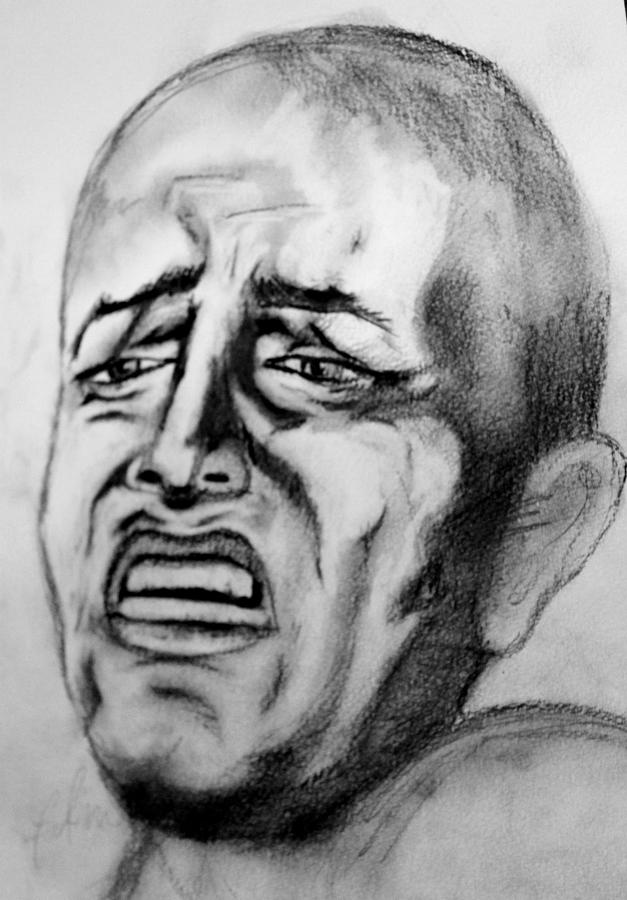The image portrays a finely detailed pencil or charcoal sketch of a black man, focusing primarily on his head, neck, and the upper left part of his shoulder. The background is an off-white or grayish hue, reinforcing the stark black-and-white palette of the artwork. The man appears to have very short hair or possibly a shaved head, with subtle stubble or a light beard around his neck and under his chin, extending to his sideburns. His face is bathed in shadows, especially around his eyes, which adds to the depth of his anguished expression.

His eyes, slightly squinted and raised towards the middle, reflect a complex blend of emotions including distress, sorrow, fear, and disgust. The dark lines and wrinkles on his face, particularly beneath his eyes, accentuate these emotions. His mouth is slightly ajar, forming a grimace that conveys a sense of impending tears or fright. His nose is pointed, and he has strong, dark eyebrows that further define his troubled look. Only his right ear is visible, with no piercings, adding to the meticulous attention to detail in the drawing. The light source appears to come from in front of him, highlighting the beautiful shading and striking contrasts. The focus on his expressive face, combined with the minimalistic and suggestive sketching of his shoulder and neck, draws the viewer's attention to the raw emotion depicted in the artwork.